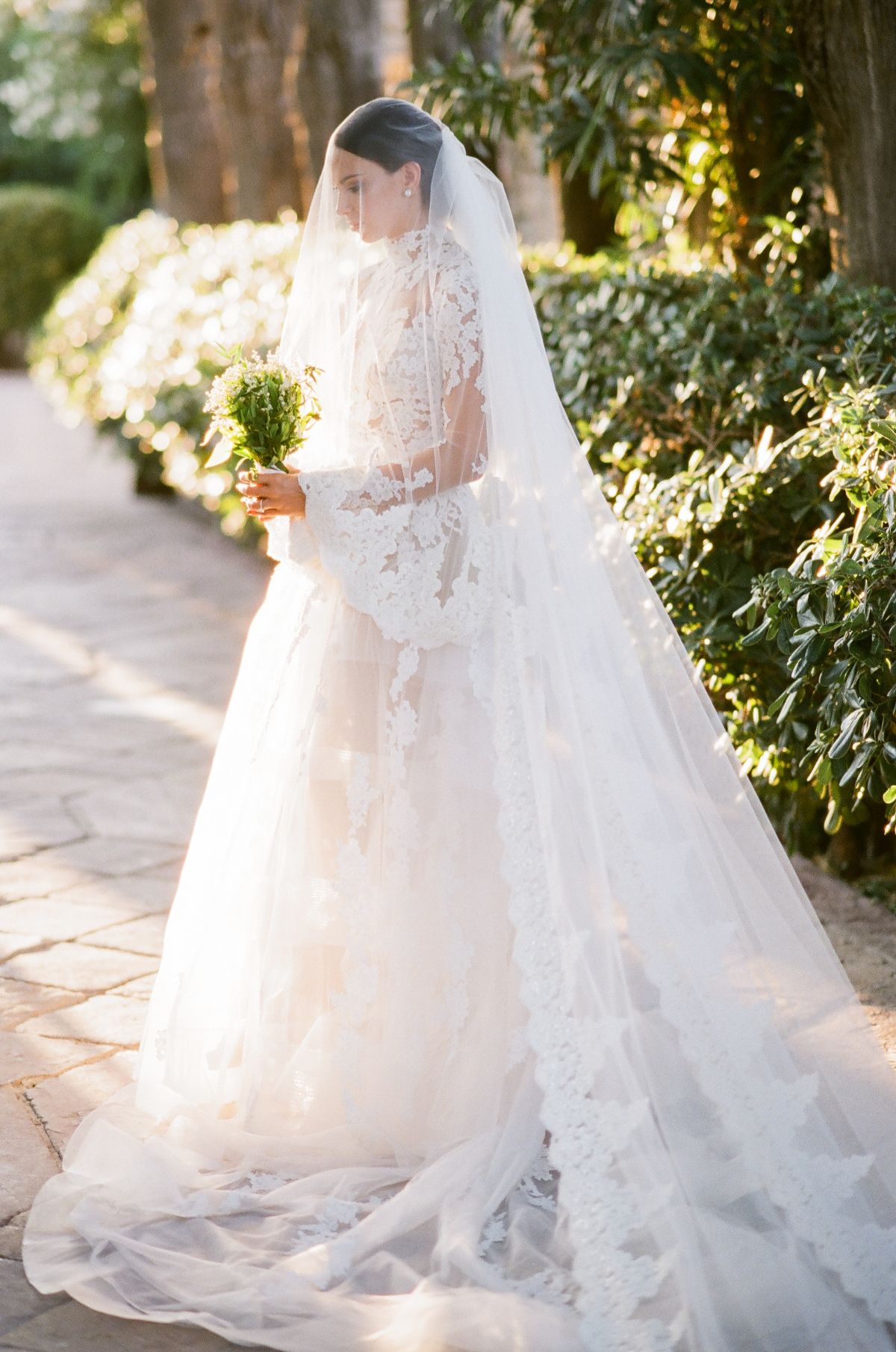This detailed photograph captures a radiant bride standing on a paved walkway as the morning sun rises, casting a gentle glow through a backdrop of towering trees—possibly redwoods—and lush greenery. The bride, posed gracefully in profile and looking to the left, is adorned in an exquisite long-sleeve white wedding gown featuring intricate lace detailing on the shoulders. Her elegant veil, adorned with lace borders, cascades over her face and extends all the way to the ground. Flowing beyond the hem of her dress, the train trails off to the bottom right corner of the image. The bride's dark brown to black hair, barely visible through the veil, complements her ensemble, which is accentuated by delicate white—possibly pearl—earrings. She clasps a modest bouquet of white flowers interspersed with greenery, mirroring the white blossoms flourishing in the shrubbery behind her. The scene, set against a clear path either at the front or back of a building, captures a moment of serene anticipation, with the verdant surroundings and emerging sunlight highlighting her bridal elegance.